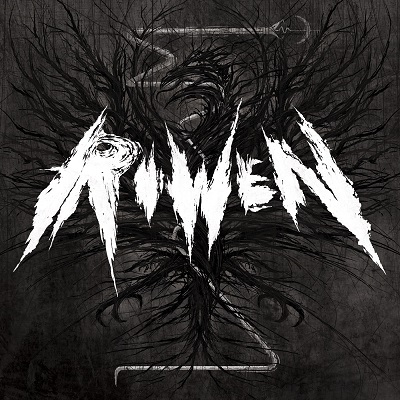This black-and-white image, potentially an album cover, features a complex and dark scene. Central to the image is a vague, dark figure that resembles a dragon or bird with indistinct outlines, its head positioned in the upper middle, facing left, and its body adorned with what appear to be feathers and possibly vine-like elements. The background is a dark gray, while a central black figure starkly contrasts against it.

Across the entire image, primitive white lettering spells out "R-O-W-E-N," with each letter appearing large and scratched, almost as if clawed into the scene. Intersecting the image are white lines that zigzag from top to bottom, starting with a sideways M shape at the top, weaving through the central figure and lettering, and sharply turning at the bottom. Despite the chaotic elements, the image remains thematically cohesive with its striking black and white contrast and primitive, almost haunting, artistic style.